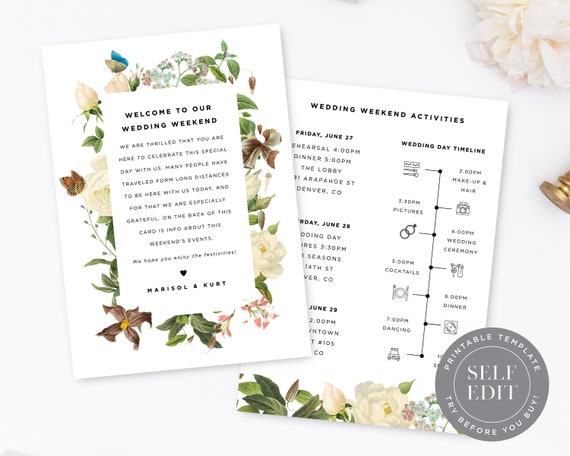This social media advertisement showcases a printable template for a wedding itinerary. The main focus is on two elegant cards placed against a light grayish-white background. Both cards feature a sophisticated design with black text on a white background. The card on the left displays a charming floral border and reads "Welcome to Our Wedding Weekend" in bold lettering, with additional details and a heart symbol at the bottom containing the names of the bride and groom. The card on the right is titled "Wedding Weekend Activities" and also includes intricate floral motifs at the bottom. Positioned slightly behind the left card, its content is divided by a vertical line with icons and text indicating different activities, though specific details are indiscernible. The scene is accented by a muted pink flower in the top right corner and a partial image of a gold cylindrical object in the middle right. Additionally, a gray circle seal in the bottom right corner highlights the features "Printable Template," "Try Before You Buy," and "Self Edit."